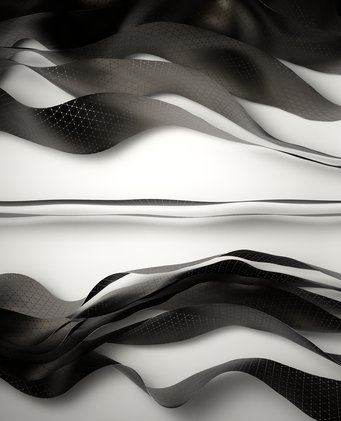This digitally created image is split into two sections, separated by a slightly wavy central line. Both sections exhibit a purely black and white color scheme, presenting a glossy, shiny appearance. The top and bottom halves, set against a white background, feature flowing black ribbons or leaves that evoke the movement of seaweed swaying underwater. The top section shows three or four long, slender, wavy leaves flowing diagonally from the left to the right, viewed from an angled perspective that reveals their thin yet wide form. The bottom section, viewed from the top, displays six similarly wavy leaves, closely clustered together. The black ribbons or leaves have a subtle pattern reminiscent of tightly combined stars and cast gentle shadows, enhancing the sense of depth and texture. The entire image is minimalistic, with no additional objects or text, making it suitable for use as a background.